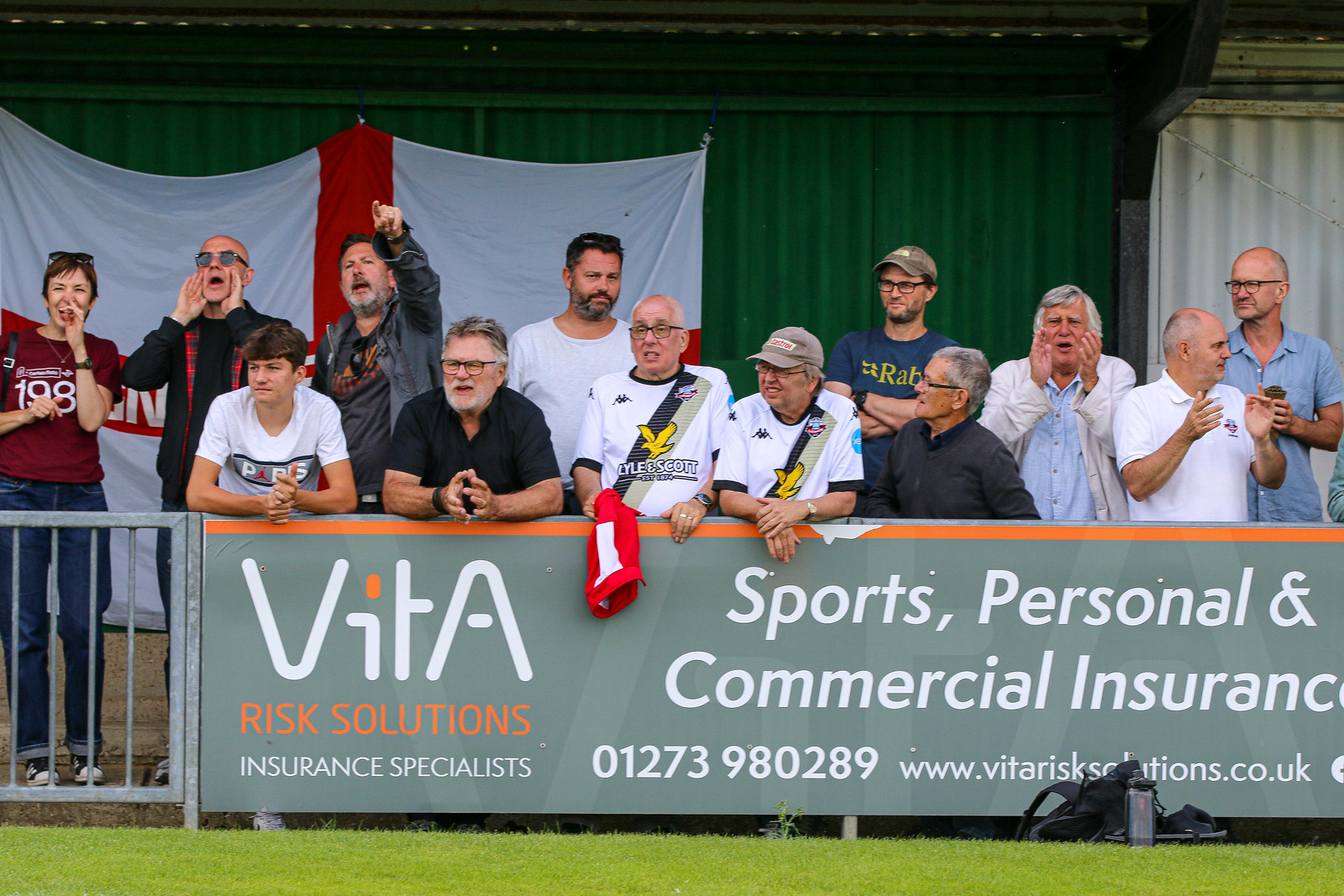In this outdoor image taken at a sporting arena, you see thirteen spectators, primarily middle-aged men, standing behind a metal railing adorned with a detailed advertisement banner. The banner reads: "Vita Risk Solutions Insurance Specialists, Sports, Personal and Commercial Insurance," followed by a phone number and a website URL (www.vitarisksolutions.co.uk). Among the group, one woman in a burgundy-red short-sleeve shirt and jeans stands out, along with a man in a blue shirt wearing a brown cap. The spectators appear to be focused on an ongoing soccer game, emphasized by the lush green grass field and green-and-white containers in the background. The attire of the individuals includes white jerseys featuring a green and black stripe, and one person in a red jersey is noticeable in the crowd. Behind them is a prominent white flag with a red cross and some green curtains or fencing, adding more context to the energetic and busy atmosphere of the scene.